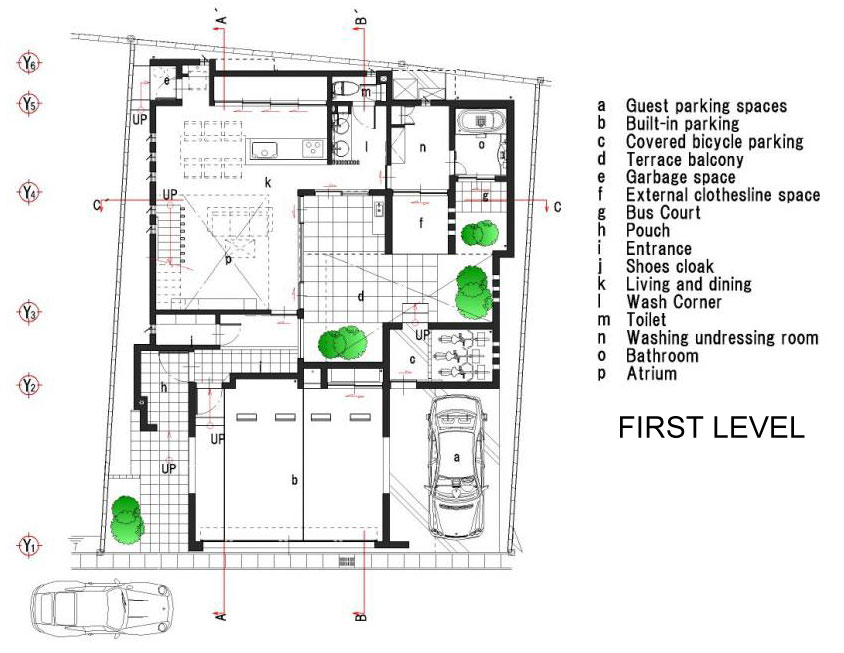This image is a detailed floor plan of the first level of a building. It is primarily black and white, with green areas designating trees and shrubs. The blueprint includes a variety of rooms and fixtures such as a sink, oven, and toilets, along with a staircase leading to an unshown second level. Two cars are depicted, one inside and one outside of the diagram. A key on the right side of the image labels various features from A to P: A is for guest parking spaces, B for built-in parking, C for covered bicycle parking, D for the terrace balcony, E for the garbage space, F for the external clothesline space, G for the bus court, H for the porch, I for the entrance, J for the shoe cloak, K for the living and dining area, L for the wash corner, M for the toilet, N for the washing and dressing room, O for the bathroom, and P for the atrium. Text below the key indicates that this blueprint represents the first level of the building.